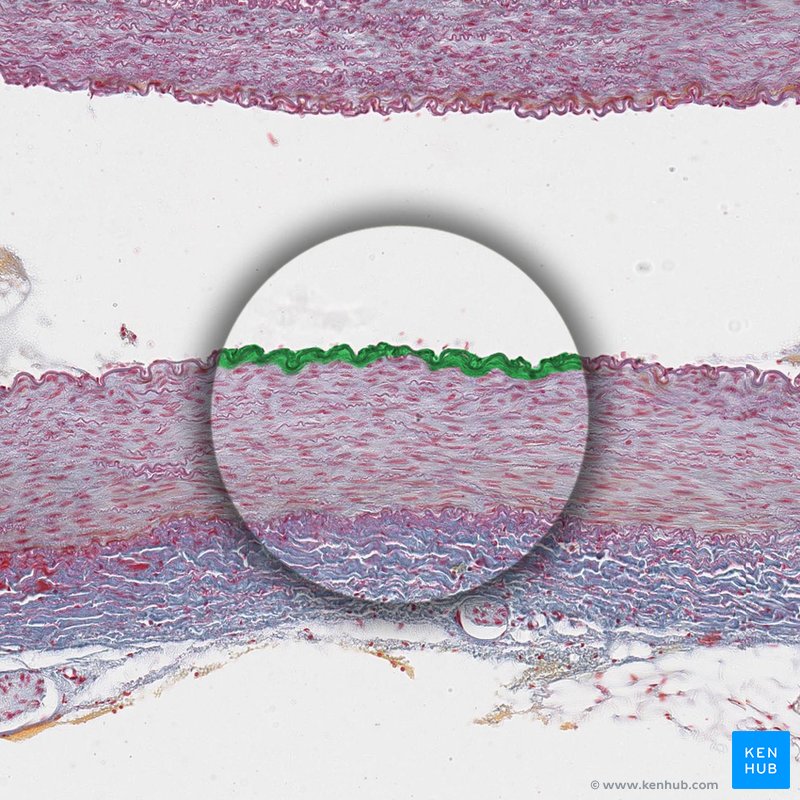The image appears to be a highly magnified view of a blood vessel or vein, showcasing a microbiological phenomenon. At the center of the image, a specific area is circled and even more magnified, drawing attention to a segment of the vessel's outer layer that is distinctly green in color. This greenish layer is estimated to be about a quarter of the total length of the depicted vessel segment, situated near the middle of the image. Surrounding this section, the remaining tissue exhibits a healthy red hue against a white background, suggesting a liquid environment. The top and bottom parts of the vessel structure are pinkish, resembling gum tissue, possibly indicating layers of flesh and veins. The image includes text reading "www.kenhub.com" and features a Kenhub logo in the lower right corner.